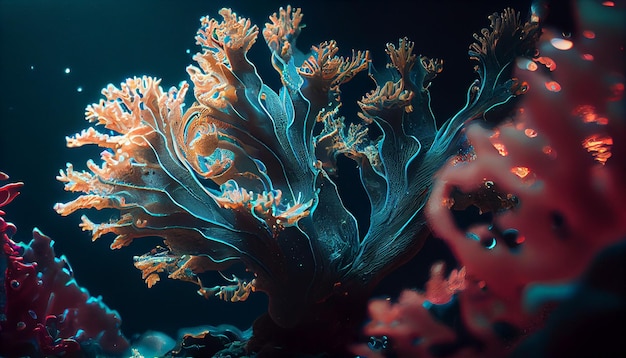This highly detailed, photorealistic digital illustration depicts an enchanting underwater scene teeming with vibrant coral life. The background is a deep, inky blue, evoking the mysterious depths of the ocean, punctuated by a few delicate pinpricks of white light and white bubbles, adding a sense of dynamic movement to the water. The main focus of the image is a striking blue-gray coral at the center, characterized by its flat, wavy planes that taper into brilliantly illuminated yellow, light orange, and ivory fringes at the tips. This coral appears shrub-like and seems to sway gently as if moved by underwater currents. 

In the lower left corner, there is a reddish-gray coral or algae, while the upper right corner features another blurred, red coral in the foreground. The blurriness here creates a depth of field that draws the eye back to the central coral. Accentuating the scene are a few pink corals adorning the left side, adding to the lush, colorful biodiversity of this underwater tableau. 

Subtle details, such as glowing white lights in the upper left and a glimpse of rocky seafloor beneath the centerpiece coral, further enrich the scene, making it a captivating portrayal of underwater coral growth.